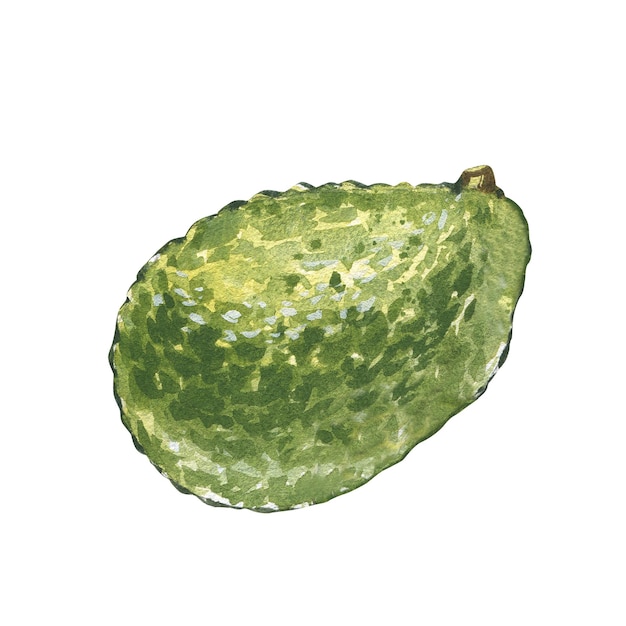This is an artistic rendering of an avocado, captured either as a drawing or a painting. The primary color is green, outlined in charcoal, with splotches of darker green and hints of light blue and yellow to suggest texture and depth. The avocado is portrayed in a side view, exhibiting a bumpy texture characterized by small pits and gentle brush strokes that give an impression of its natural skin. At the top, there is a small brown stem that barely protrudes from the fruit. Reflective elements in the painting include spots of lighter colors, including white, indicating a glossy or sunlit surface. This piece emphasizes the detailed, multi-tonal surface of the avocado, creating a vivid and tactile representation.